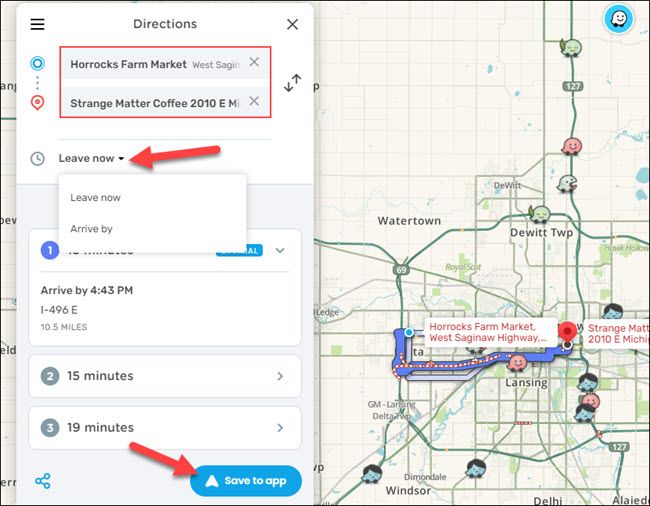Screenshot of a navigation app, possibly resembling an open-source service, showing a detailed map of central Michigan, highlighted areas labeled Watertown, DeWitt Township, Lansing, Windsor, and Delhi. The map includes whimsical elements like green and pink emoji-like figures scattered across the region, resembling characters from games like Pokemon or Pac-Man.

Highlighted within the map are two specific locations: Horrocks Farm Market on West Saginaw Highway and Strange Matter Coffee. A route is traced between these two points, marked clearly on the map. An overlay window at the top right summarizes the route options, with choices such as "Leave Now" or "Arrive By" for planning the journey. 

Further details show a specific travel option: arriving by 4:43 PM via I-496 E, covering a distance of 10.5 miles. The image is annotated with red arrows; one pointing towards "Leave Now" option and another towards a "Save to App" button at the bottom, indicating specific user interactions for ease of use.